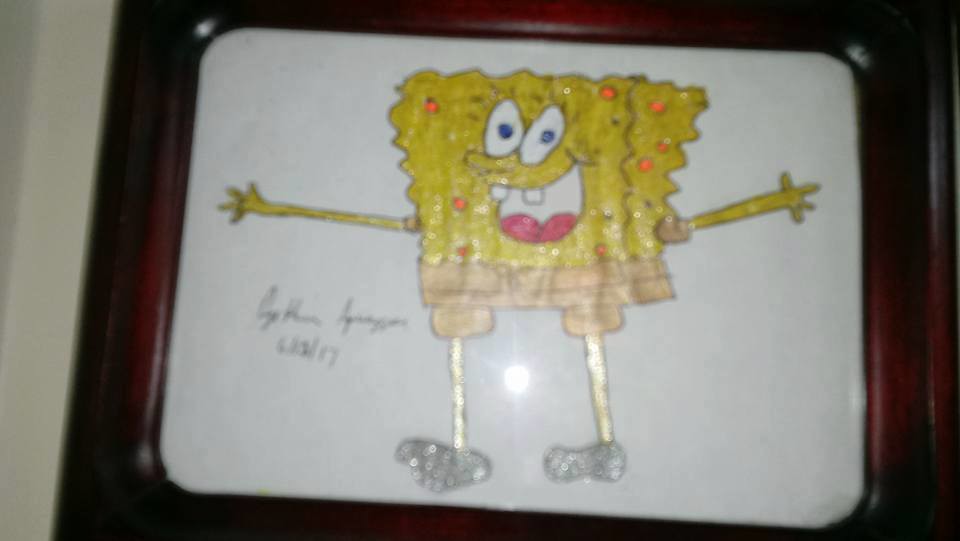A slightly out-of-focus, amateur drawing of SpongeBob SquarePants, rendered on a small whiteboard with a black rim, hangs on a door. The whiteboard is secured to the door, which has white walls and door panels visible around it. SpongeBob is depicted with his arms extended horizontally and his iconic spindly legs and square pants. The drawing, although not of professional quality, is instantly recognizable due to SpongeBob's distinctive features. The artwork appears to be signed in cursive, possibly with the name "Cynthia," though the signature is difficult to decipher. A date, which looks like 6-12-17, is also present but hard to read. There is a noticeable reflection from a flash between SpongeBob's legs, creating a bright hotspot on the image.